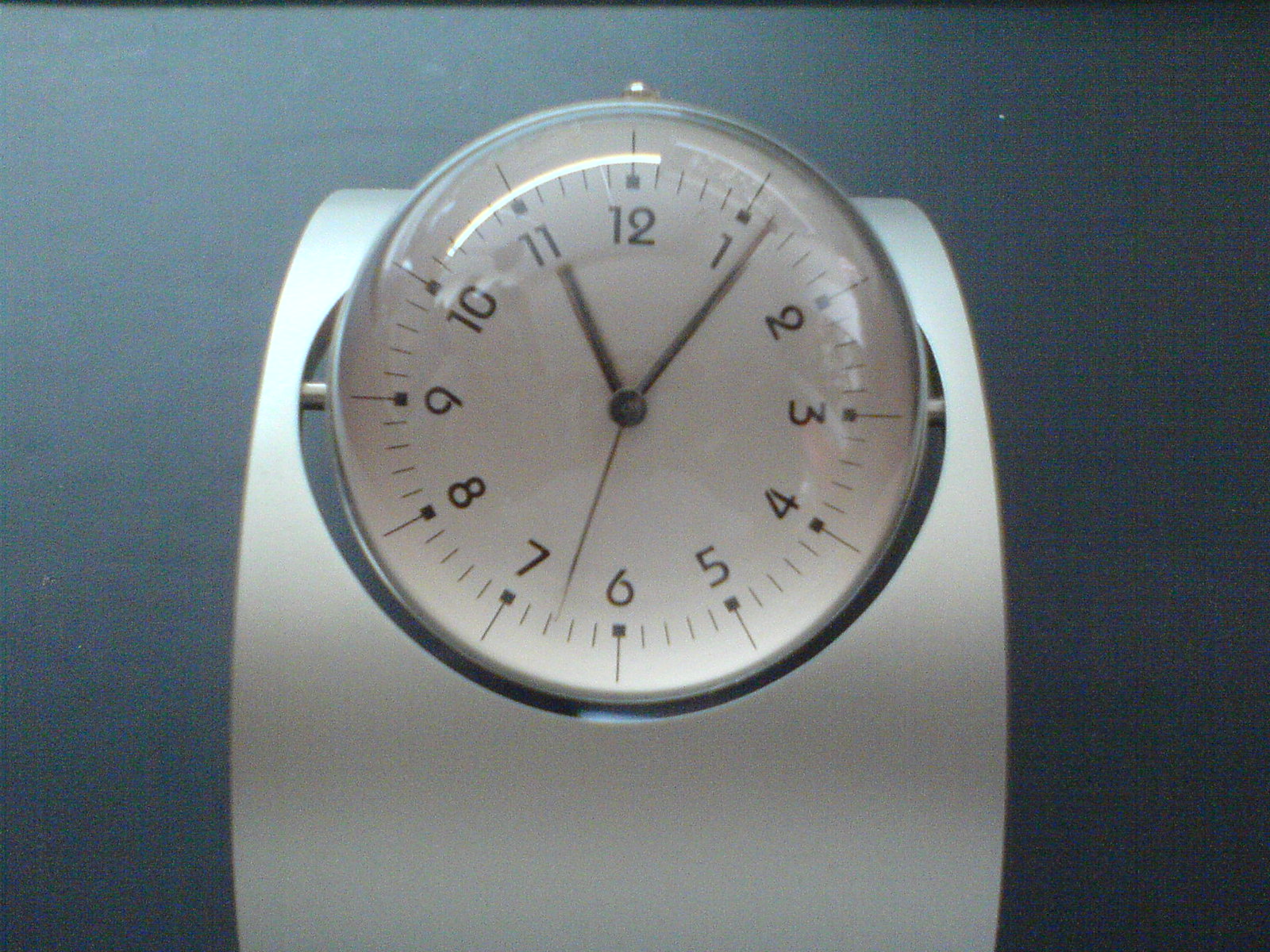The photograph features a minimalistic, old-fashioned clock with a white face and black numerals, designed for a traditional reading with hour, minute, and second hands. The clock, which may also be interpreted as a watch, is supported by a sleek, silver or white stand, giving the appearance that it is hovering in mid-air due to its rotating hinge mechanism housed within a small cavity of the base. This mechanism allows the clock face to be adjusted to various angles. The glass cover over the face is bulbous and dome-shaped, reflecting light like a water droplet. The hands indicate a time of 11:06, with the little hand at the 11 and the big hand just past the 1, while the second hand lies between the 6 and the 7. The entire setup sits against a medium blue-gray background, and there is a small stainless steel button at the top of the clock, probably for adjusting the time or setting an alarm. There is no branding visible on the clock, suggesting a clean and functional design, suited perhaps for an eBay-style listing.